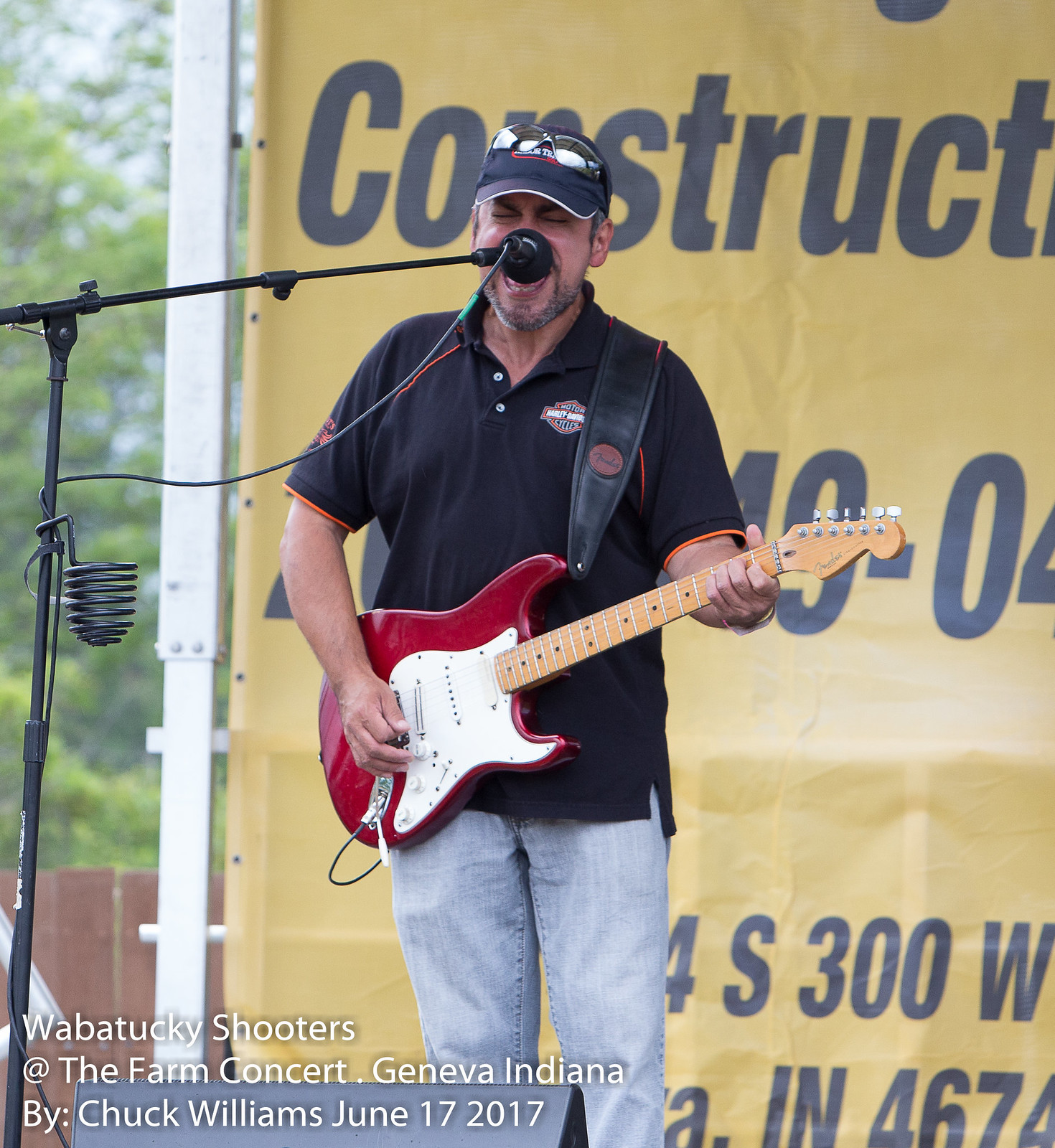A vibrant snapshot captures a passionate moment during a live performance. A man is center stage, immersed in his musical rendition as he strums a red electric guitar adorned with white trim. Mid-song, he leans into a microphone affixed to a stand, singing with fervor. His attire reflects a rugged style: a shirt emblazoned with the iconic Harley Davidson motorcycle emblem and a black cap, upon which a pair of sunglasses rest. In the background, a banner partially visible reveals details such as the word "construction," an address, and a phone number. At the bottom left corner, text provides context: “Wabatuckee Shooters at the Farm Concert, Geneva, Indiana, by Chuck Williams, June 17th, 2017.” The scene encapsulates the raw energy and enthusiasm of live music, set against the backdrop of a rustic concert venue.